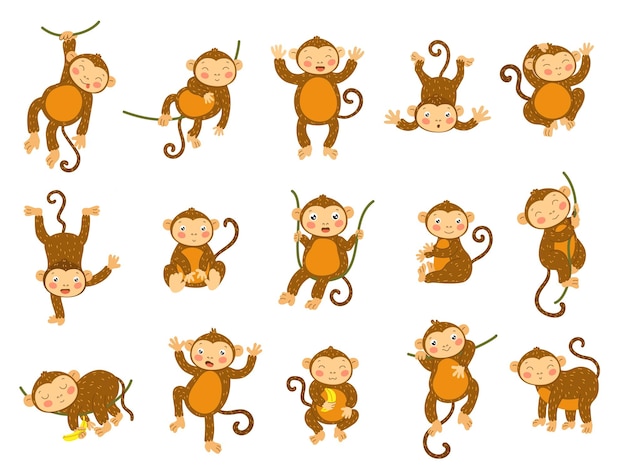The image depicts a delightful cartoon illustration featuring 15 playful monkeys arranged in three rows of five on a white background. Each monkey, characterized by medium brown fur, curly tail, pink rosy cheeks, and an orangish belly, displays a distinct and expressive face. The monkeys are shown in various humorous and dynamic positions: one hangs from a vine, another sits on a vine, one raises its hands in the air as if cheering, while another appears to have fallen over. Additional antics include a handstand, jumping, swinging, sitting pensively, dancing, and eating a banana. These evenly spaced, charmingly detailed illustrations capture the monkey in different stages of activity, from sleeping to laughing, all showcasing its joyful and spirited nature.